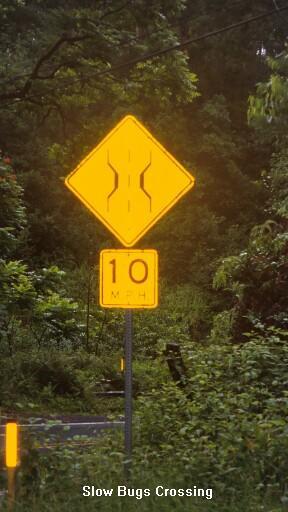In this vibrant image, a prominent yellow sign catches the eye, set against a lush background of green leaves and plants. At the very bottom of the sign, the words "Slow Bugs Crossing" are displayed horizontally in white lettering. To the left of this sign, a smaller yellow sign is visible, adding to the layered arrangement. Toward the center-right of the image, a gray pole emerges, supporting a square sign that indicates "10 MPH," though the letters 'P' and 'H' appear considerably faded. Above this square sign, there is a yellow diamond-shaped sign featuring two vertical lines that branch out symmetrically to the left and right, forming a path-like pattern. In the distance, a glimpse of a gray road is visible, merging seamlessly into the backdrop dominated by the verdant canopy of leaves and a few black telephone wires stretching across the upper portion of the frame. The entire scene exudes a sense of serene natural beauty interspersed with subtle urban elements.